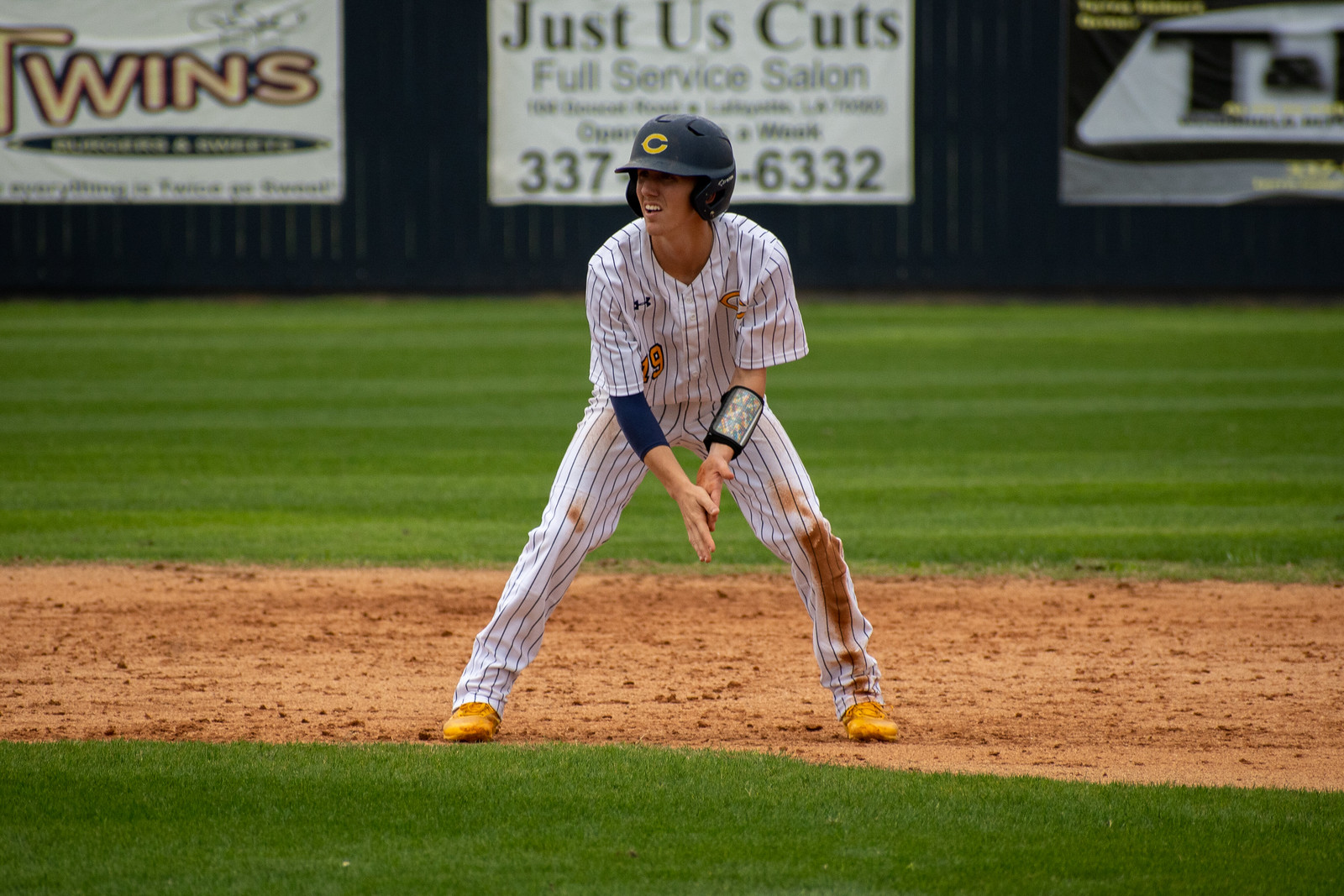The image depicts a teenage or high school baseball player standing on the sandy dirt portion of a baseball field, with lush green grass and a blue fence in the background. The player is dressed in a classic white jersey and pants with blue stripes, complemented by yellow shoes. He is wearing a navy blue helmet featuring a yellow 'C' emblem. Notably, there is a dirt stain running from his left knee to his ankle. On his arm, he has an armband similar to those in football, typically used for play calls. The ground beneath him appears either red or muddy. In the blurred background, various advertisements are partially visible on the blue fence, including a prominent sign for "Just Us Cuts, Full Service Salon, 337-6332" and another indistinct one for "Twins."